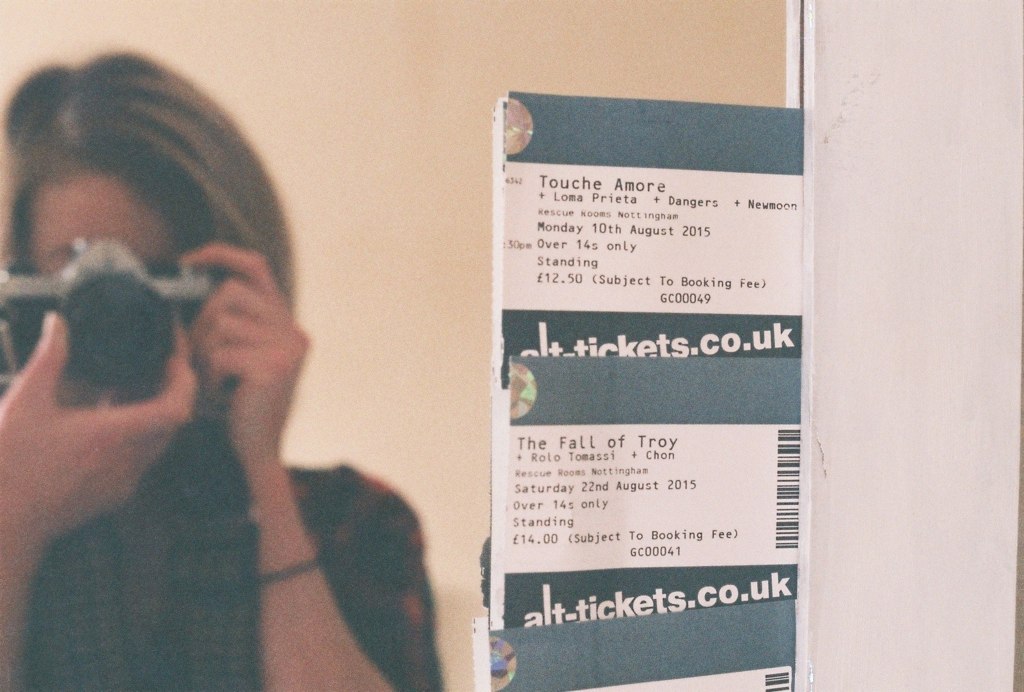A woman with black-to-light-brown ombre hair, parted on the left, is capturing her reflection in a mirror using a camera. The camera has a black center with a silver casing, and in her right hand, she holds it steady with her fingers poised over the button. Her left hand supports the lens, thumb touching the lens, and other fingers on the opposite side. She wears a dark plaid shirt and a black bracelet on her right wrist. Behind her are peach-colored walls with a piece of paper tucked into the mirror's seam. This paper displays details of two events: "Touche Amore at Loma Prieta, Dangers, Newsroom, Rescue Rooms, Monday, August 10, 2015," and "The Fall of Troy, Rolo Tomassi, Chon, Saturday, August 22, 2015." Both events are noted as "Over 14s only," with the first event costing £12.50 and the second £14, each subject to a booking fee, and available through alt-tickets.co.uk. The wall to the right of the photograph, visible in the reflection, is white plaster with some visible cracks where it meets the mirror.